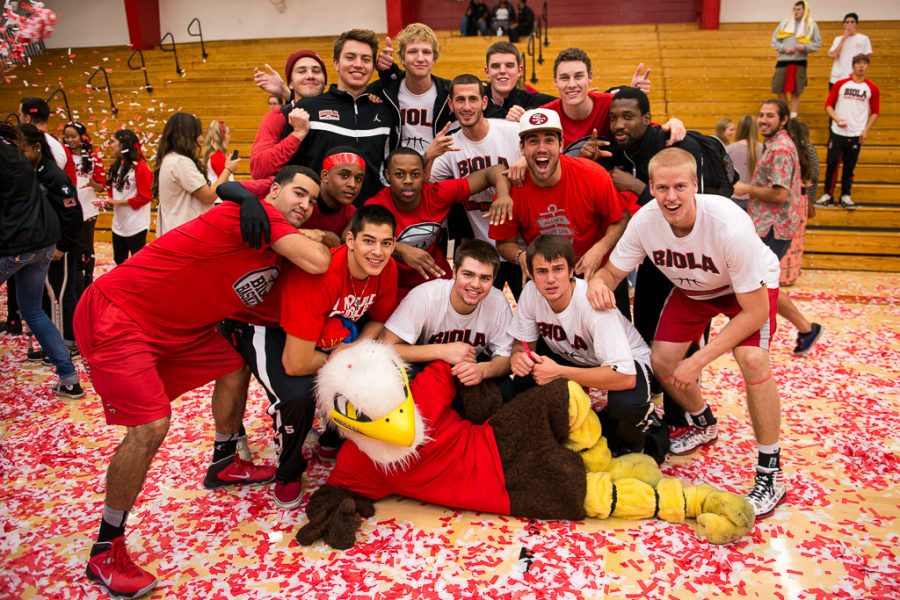The photograph captures a jubilant scene inside a school gymnasium following a sporting event. In the center, a group of people, likely a mix of players and fans, are celebrating amidst a sea of red and white confetti scattered across the gym floor, which is partially visible beneath the colorful fragments. Dominating the foreground is the school mascot, a regal eagle with a white head, yellow beak, and yellow eyes, dressed in a red shirt and brown shorts, laying down amidst the commotion. Surrounding the mascot, participants in the celebration are clad predominantly in red, white, and black attire, with some sporting red and white uniforms accented with black. The gym's background features rows of brown bleachers with more people—some seated, some standing—engaged in their own activities, adding to the lively atmosphere. The red and white décor above the bleachers enhances the sense of school pride and unity in the image.